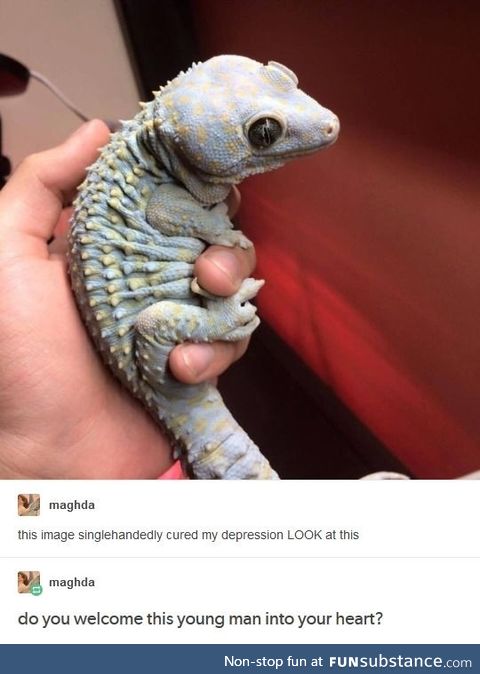A vividly colored image shows a light green and light yellow iguana, with hints of bluish-gray on its body, being gently held in a man's hand. The iguana's large, black eyes with vertical slits and round yellow specks along its snout and body are striking against the warm brown background. Tiny claws are wrapped delicately around the man's fingers, and its tail extends out of the frame. Underneath the image, two enthusiastic captions from a user named Magda read, "This image single-handedly cured my depression. Look at this!" and "Do you welcome this young man into your heart?" A blue banner at the bottom credits the image to "nonstopfun at funsubstance.com."